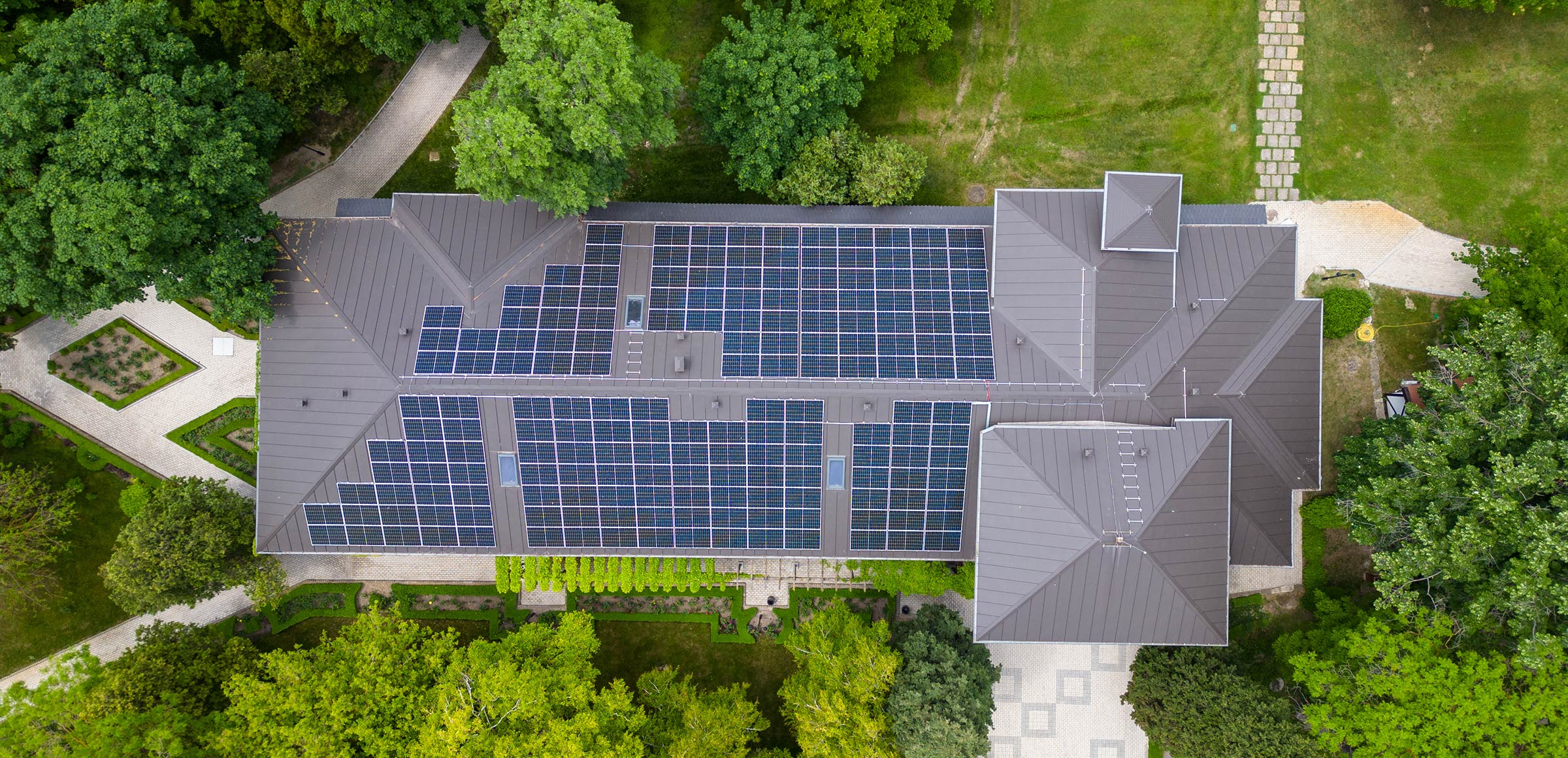The image shows a bird's-eye view of a multi-floored, A-frame house with a gray metal roof adorned with numerous blue solar panels arranged in a grid pattern. The solar panels cover most of the left side of the roof, stopping at various angles to match the roof's structure, while the right side features fewer panels and several protruding points. The house is surrounded by dense, dark green vegetation and some grassy areas, suggesting a springtime setting. Various walkways extend from the house, including a light cream-colored path with decorative gray squares and a cobblestone walkway. The house is centrally located within the image, emphasizing its rectangular shape amidst the verdant landscape.